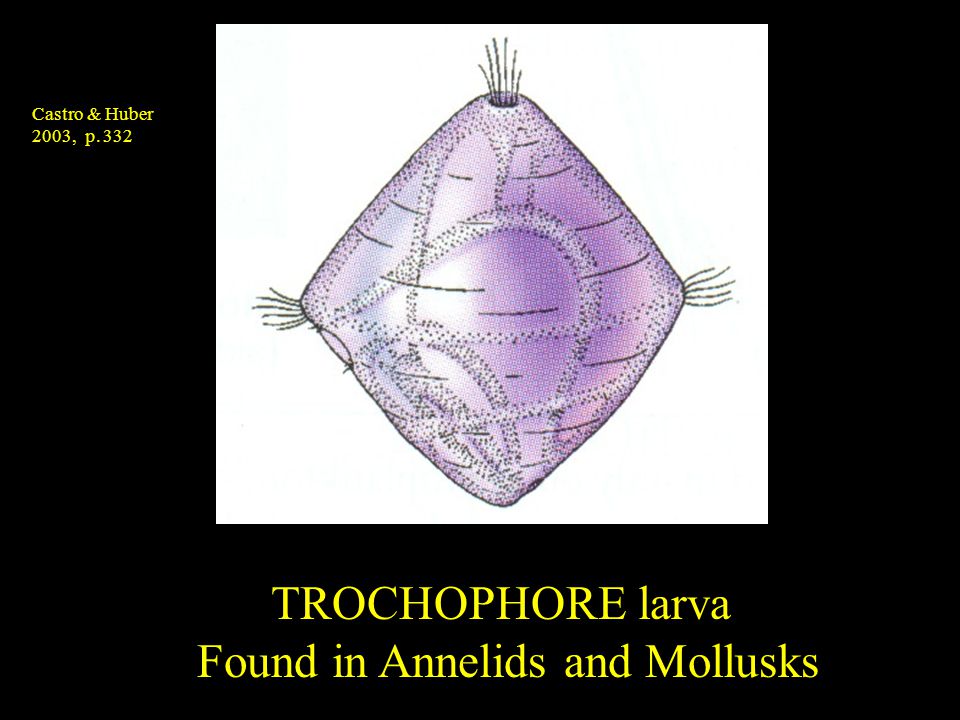The image prominently features a detailed, digitally rendered depiction of a diamond-shaped trochophore larva, characterized by its purple and white hues and fine hair-like structures extending from the ends. The central image is set against a bright white background, which contrasts starkly with the overall black background of the rectangular slide. In the top left corner, yellow text reads "Castro and Huber, 2003, page 332," indicating the source of the information. At the bottom, also in yellow text, is a caption that identifies the larva as being found in annelids and mollusks, reinforcing its educational purpose. This slide appears to be a part of an educational poster or presentation, designed to visually convey specific biological information.